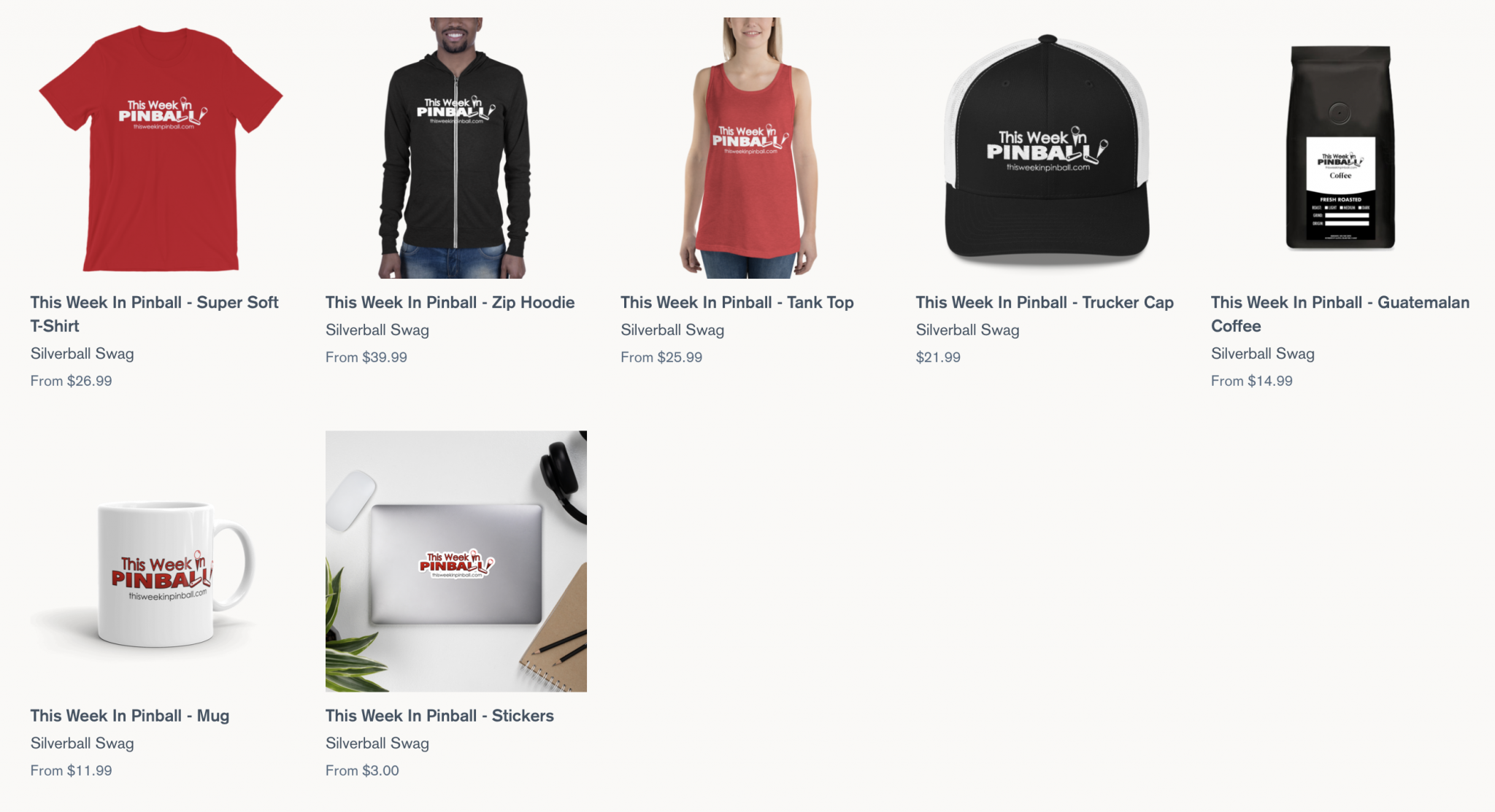This image is a cropped screenshot showcasing a webstore page featuring a variety of branded products. The layout includes seven product thumbnails organized in two rows. The first row displays five items: 

1. A vibrant red t-shirt sporting the “This Week in Pinball” logo prominently on the front. The product title, "This Week in Pinball Super Soft T-Shirt," is displayed in bold, black font, accompanied by the price beneath it.
2. A stylish zip-up hoodie bearing the same “This Week in Pinball” logo, with the starting price listed as $39.99.
3. A women’s tank top also featuring the “This Week in Pinball” logo.
4. A cap embroidered with the “This Week in Pinball” logo.
5. A bag of Guatemalan coffee, complete with the “This Week in Pinball” logo on the packaging.

The bottom row contains two additional products:

1. A mug adorned with the “This Week in Pinball” logo.
2. A sticker featuring the same logo.

Each product image is detailed and clearly showcases the “This Week in Pinball” branding, providing potential buyers with a vivid preview of each item.